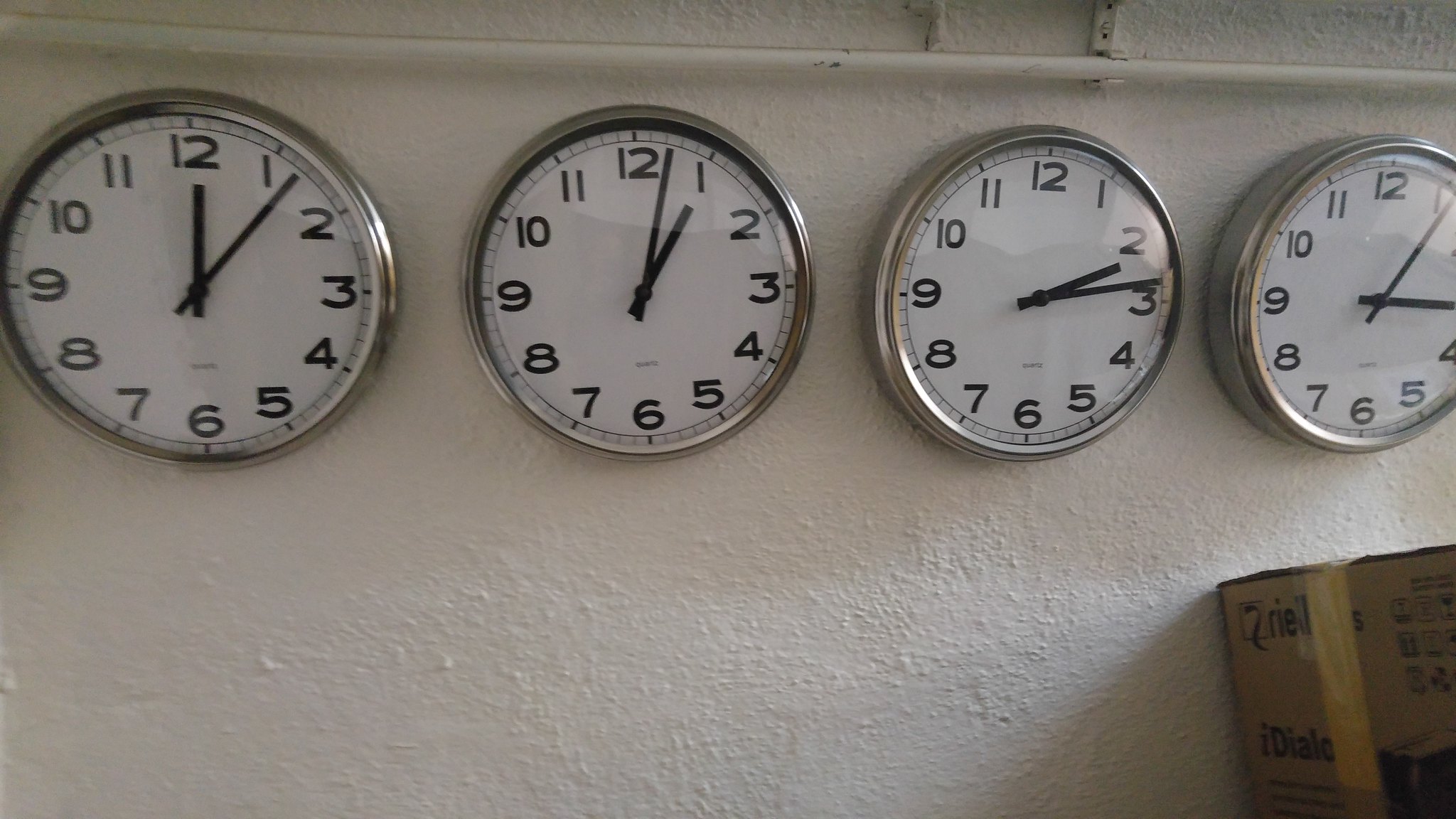In the photograph, a white rendered wall is adorned with four circular clocks arranged in a row. Each clock is encased in a silver housing with white faces, black numeric digits, black hash marks, and black hands. The first clock shows the hour hand at 12, and the minute hand approximately 7 minutes past the hour. The second clock indicates a time of about 2 minutes past 1 o'clock. The third clock displays a time around 14 minutes past 2 o'clock, and the fourth clock, slightly cut off, reads just past 3 o'clock. Above the clocks, a horizontal cylindrical white pipe or some form of piping is visible. Near the bottom right corner of the image, a stack of dark brown cardboard boxes is seen, identifiable by black text and a piece of yellow tape over them, contributing to the scene's utilitarian atmosphere.